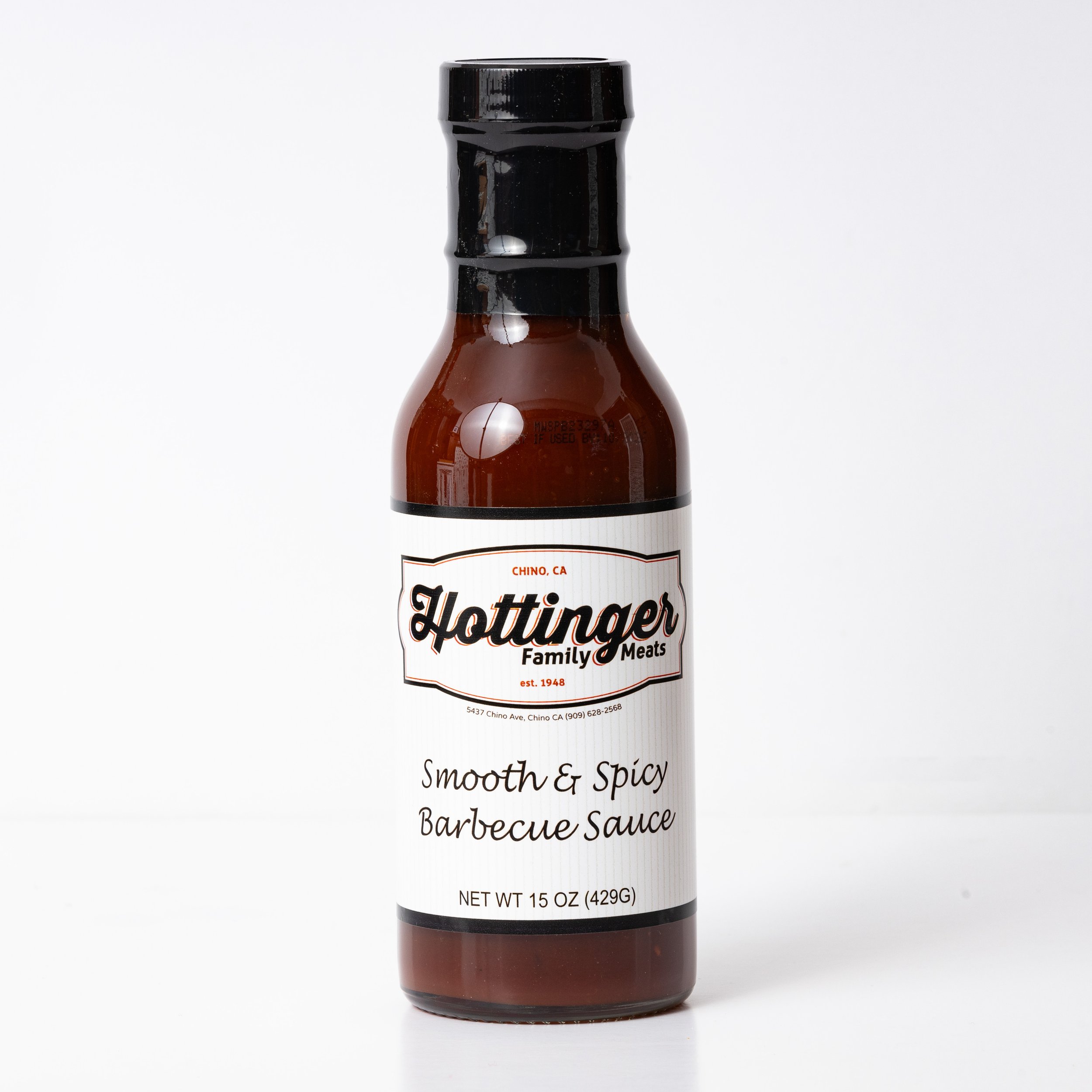This image features a tall, sleek glass bottle of barbecue sauce set against a white background, casting a shadow on the surface below. The bottle is sealed with a black plastic band around the neck and lid. The transparent glass showcases the dark red barbecue sauce inside, which contrasts sharply with the simple, white label that wraps around the center of the bottle. The label is adorned with black and red fonts, stating "Chino, California" and "Hottinger Family Meats," established 1948. "Smooth and Spicy Barbecue Sauce" is written below, indicating a net weight of 15 ounces (429 grams). The words "Hottinger" are elegantly scripted in cursive, while "Family Meats" is presented in a sans serif font, reminiscent of Arial. Subtle reflections on the top half of the bottle hint at lights positioned in front of it.